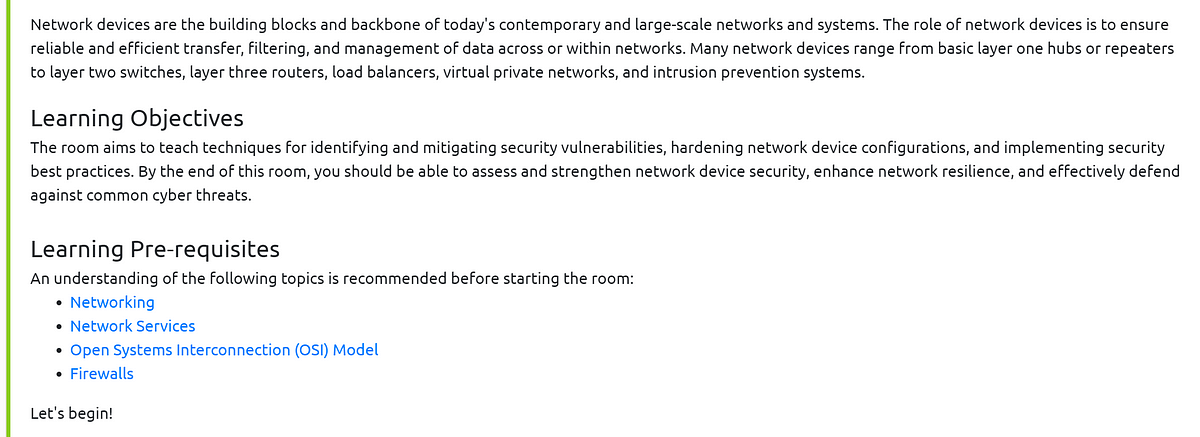The webpage features an introductory paragraph on its homepage, framed by a green border accentuated with a subtle beige outline that blends with the page's overall background. The paragraph begins by stating, "Network devices are the building blocks and backbone of today's contemporary and large-scale networks and systems." It elaborates on the critical role of network devices in ensuring reliable and efficient data transfer, filtering, and management across or within networks. The text explains that these devices range from basic Layer 1 hubs and repeaters to Layer 2 switches, Layer 3 routers, load balancers, Virtual Private Networks (VPNs), and Intrusion Prevention Systems (IPS).

Directly beneath this paragraph, in bold black letters, is the heading "Learning Objectives." It outlines the goals of the module, which include teaching techniques for identifying and mitigating security vulnerabilities, hardening network device configurations, and implementing security best practices. By the end of the module, participants should be capable of assessing and strengthening network device security, enhancing network reliability, and effectively defending against common cyber threats.

Below the learning objectives, the section "Learning Prerequisites" advises that an understanding of networking, network services, the Open Systems Interconnection (OSI) model, and firewalls is recommended before proceeding. These prerequisites are listed in blue text for emphasis.

At the bottom of the page, the phrase "Let's begin" is prominently displayed in black, signaling the start of the learning journey.